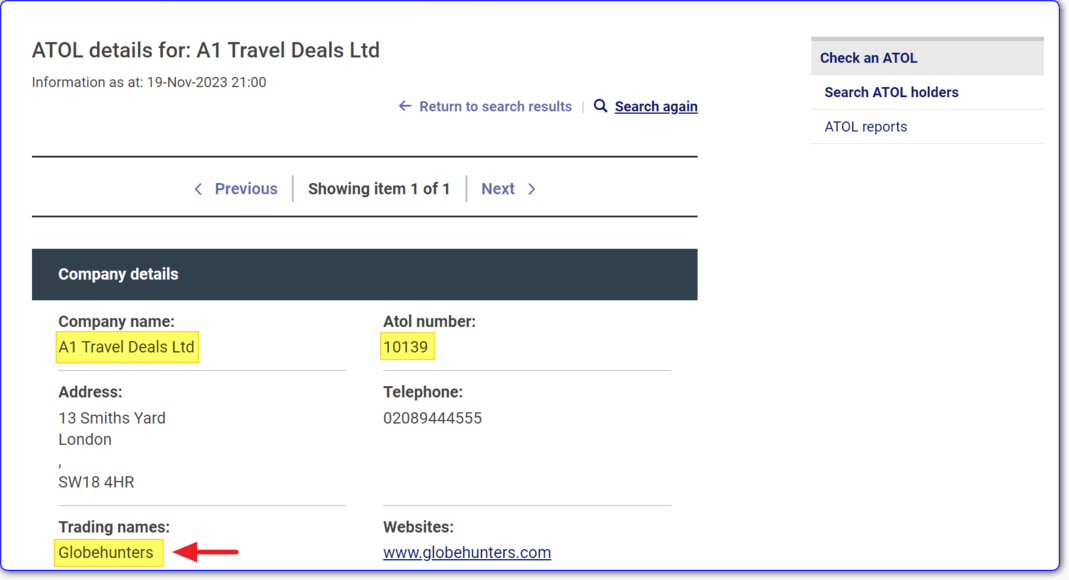A detailed screenshot with a white background prominently displays the text "ATOL" in capital letters over a gray rectangle. This image provides various details for "A1 Travel Deals, LTD," including a check-in for ATOL compliance. At the top, multiple navigational options are visible: "Search ATOL Holders," "ATOL Reports," and "Information as at 19 November 2023, 21:00."

On the left side of the screenshot, there is a left arrow and the text "Return to Search Results," followed by a right-facing magnifying glass icon alongside the text "Search Again." Below this, navigational buttons display "Previous" and a left arrow, indicating "Item 1 of 1," as well as "Next" with a right arrow.

In the middle of the image, a blue rectangle with white text reads "Company Details," and highlights the company name, "A1 Travel Deals, LTD," in yellow. The company’s ATOL number, also highlighted, is "ATOL 10139." Additional company details include the address, "13 Smiths Yard, London, SW18 4HR," and a telephone number, "020 8944 4555."

Lastly, under the address, the trading name "Globe Hunters" is highlighted in yellow with a red arrow pointing to it, emphasizing its significance in the provided information.